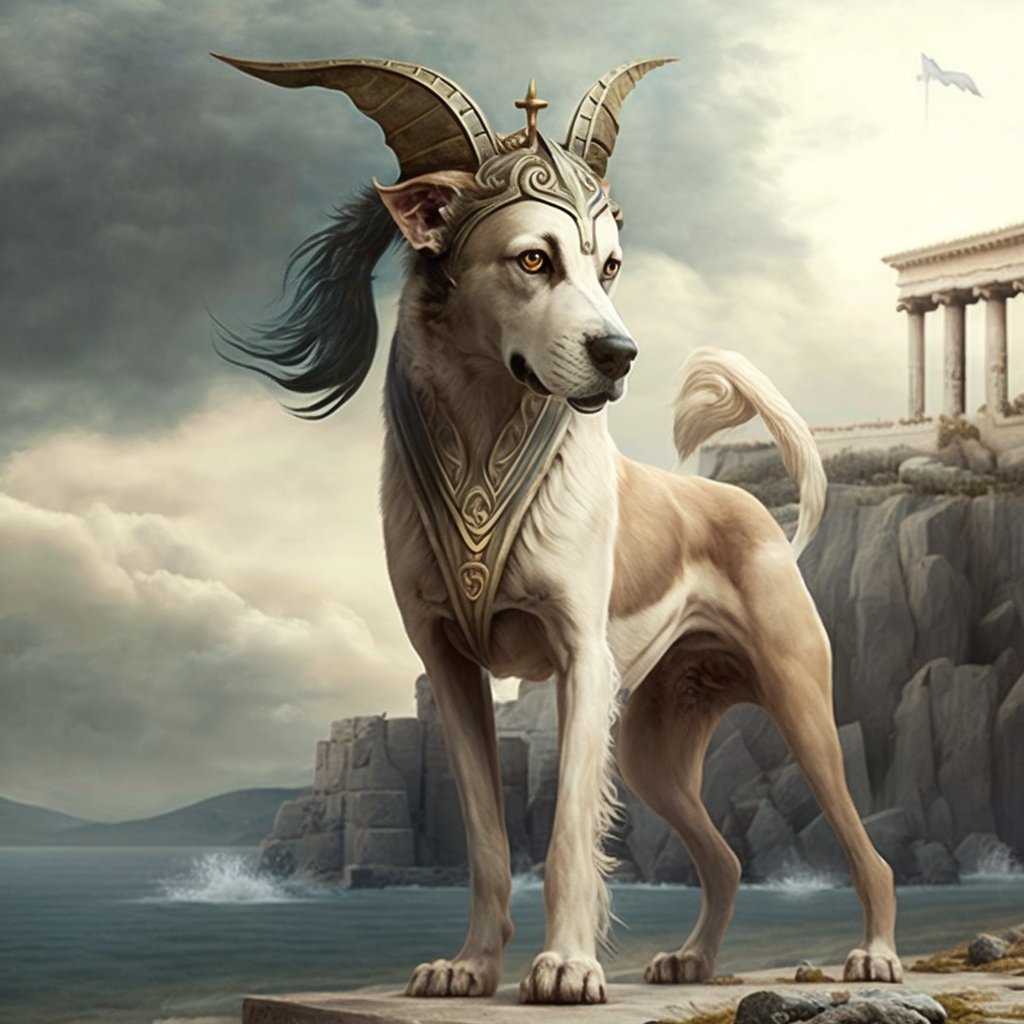This detailed painting portrays a tall, slender dog standing proudly on a concrete or stone slab. The dog, a mix of white and merle coat with brown patches and black hair, exudes a regal presence with a tail up in the air and a fluffy tip. The front legs are notably thin and slender, bearing a fur texture. Around the neck, the dog wears a metal collar that descends into a V-shaped chest plate, resembling medieval armor, enhancing its warrior-like appearance. 

Adding to its majestic look, the dog sports a medieval helmet, dark gray metal with wing-like appendages on top, and a cross adorning the front. The helmet extends down between the eyes and features what appears to be a feathery mane or tail emerging from the back, enhancing its fierce yet noble demeanor. 

In the background, a scene reminiscent of ancient Greece unfolds, with a towering cliff of both natural and man-made rocks leading up to Greek pillars and cement structures that evoke the grandeur of Athens. To the dog's left, a river flows by, with waves splashing onto the rocky shoreline. Above, puffy and dark clouds loom, creating a dramatic sky.

Every element combines to create a vivid image of a warrior dog amidst a grand ancient landscape, evoking strength, pride, and historical resonance.